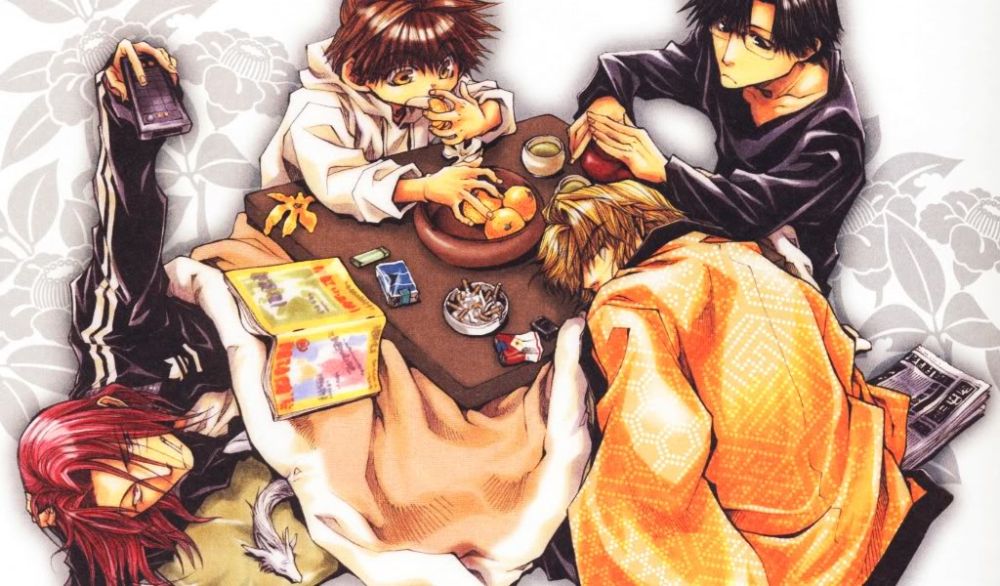The image is an intricately detailed manga-style illustration depicting a scene of four young individuals around a square coffee table. Prominently featured is a character with long reddish hair, partially covering their face, wearing a black Adidas-style track jacket with white stripes, and holding a phone as if attempting to take a selfie. This person is also covered with an orange blanket, and a whimsical small dragon-like creature peeks out from beneath it. On top of the blanket rests a large piece of wood or table, and a book is propped on top. The individual appears slightly annoyed, possibly trying to watch television.

Flanking this person on either side are two more characters. On the left side of the table, a child with a concentrated expression is reaching into a bowl of fruit, presumably picking an orange. Opposite them, another teenager with shoulder-length hair and rectangle glasses frowns as they rest their elbow on the prone person at the table. This third individual lies face down, their hair cascading over their face, and is also enveloped in an orange blanket or jacket. 

Seated near the feet of the prone individual, the fourth character appears to be polishing an apple, also contributing to the subdued mood, as no one looks particularly happy. The table itself is cluttered with various items, including an ashtray brimming with cigarette butts, several cigarette packs, a lighter, and a bowl of fruit. The floor beside the table is strewn with newspapers. Behind the group, the backdrop features a black and white floral print, completing the image's detailed and somewhat melancholic ambiance.